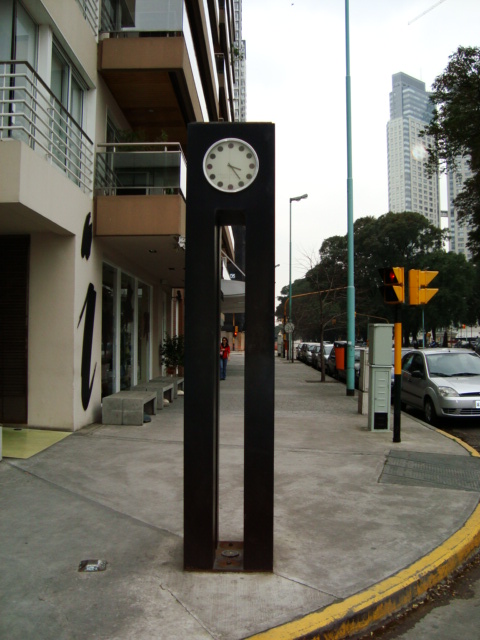This is a color photograph taken during daytime, depicting a city street scene dominated by a distinctive art installation-like clock. The clock, with its white face and dot-marked numbers, reads approximately 3:25 PM against a backdrop of a cloudy sky. The clock is positioned high atop two long, black metal legs that give it a striking, sculptural Art Deco aesthetic, almost resembling a figure standing upright.

This scene unfolds on a sidewalk that curves gently in the foreground. To the right side of the frame, several cars are parked, including a gray car and a red car, next to what appears to be an apartment complex or condos. A notable feature on the building's wall is a painted eye-like dot, purposefully designed rather than graffiti. The sidewalk curves around a worn and dirty yellow-painted curb. Off in the distance, looming skyscrapers can be seen, providing a backdrop to the street scene. A red traffic light is also visible, signaling the bustling urban environment.

One person can be seen in the distance on the sidewalk, which runs parallel to a large building that stretches the length of the view on the left. The clock mounted on its stylish pillars serves as a focal point, captivating passersby amidst the ordinary city surroundings.